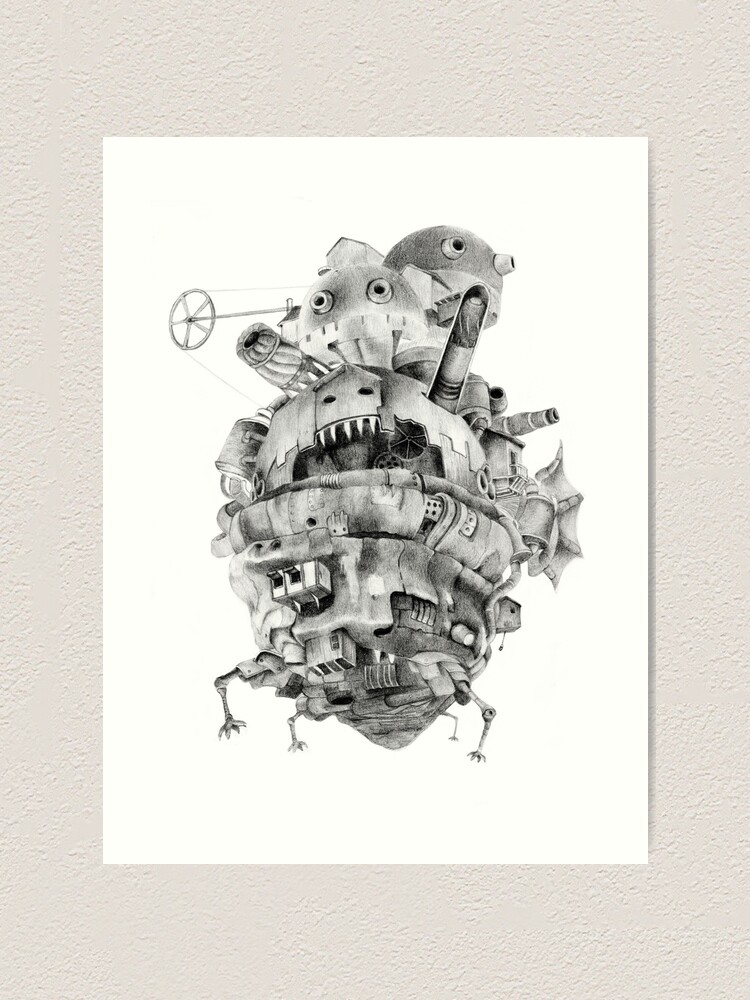The image features a black and white, intricate pencil drawing set against a white background with an off-white border. Central to the composition is a large, fantastical structure resembling a chaotic conglomeration of robot heads and mechanical components. The structure is characterized by a beehive-like shape with numerous windows and jagged teeth, giving the impression of sentient, bulging eyes looking in various directions. Protruding from the base are four metallic legs, suggesting mobility. Additional details include thin, cannon-like appendages extending from the sides and fin-like structures that evoke a sense of both architectural complexity and industrial design. The entire piece exudes a whimsical yet eerie mechanical aesthetic, blurring the lines between a house and a menacing robotic entity.